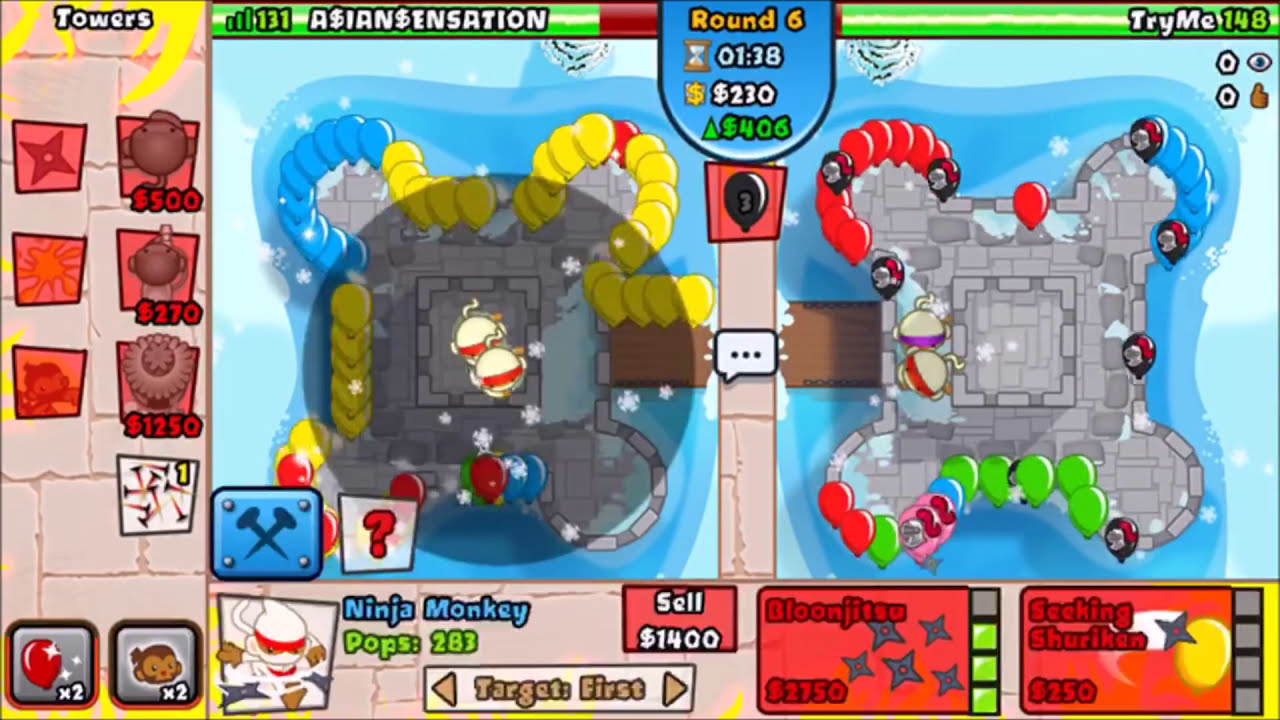The image appears to be a vibrant, busy screenshot of a video game, featuring two concurrent games displayed side-by-side. The left section of the image shows a vertical interface with gray rectangular tiles topped by six red squares, each containing icons and cash amounts in red text outlined in black ($500, $270, $1,250). This section is labeled "TOWERS" and includes additional tiles at the bottom depicting a red balloon and a brown monkey, both labeled with "times two". 

In the main gameplay area, there are two castles, each surrounded by blue moats and brown drawbridges, viewed from an overhead perspective. Numerous colored balloons in shades of blue, yellow, red, green, and pink, along with white and red bombs, populate the space around the castles. The top section displays green bars with the usernames "Asian Sensation" on the left and "Try Me" on the right, indicating the two players participating in the game. 

Additionally, the bottom part of the image shows more text and graphics, including a ninja character in a white suit labeled "Ninja Monkey Pops 283" accompanied by throwing stars and other icons. The interface is further adorned with various numerical values and progress indicators, all contributing to the overall complexity of the game's visual presentation.